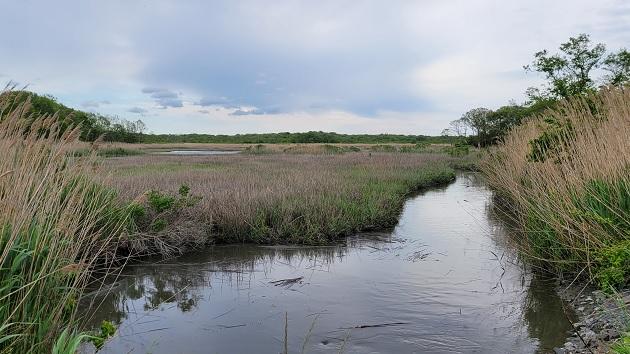In this serene image, we see a vibrant wetland landscape featuring a dynamic blend of lush green grasses and tan reeds, which grow abundantly out of the clear, clean water. The water appears to be gently flowing, reminiscent of an inland waterway or bayou, possibly concealing a deeper current. Rocks or gravel line the water's edge on the right, adding texture and variety to the scene, while a hill and a distant tree line anchor the horizon. The day is marked by a clear sky with a few scattered clouds, creating an inviting and tranquil atmosphere perfect for fishing or observing wildlife such as fish, white water birds, or potentially even reptiles. Every element, from the green and brown vegetation to the clean and clear water, combines to paint a picture of natural beauty and stillness.